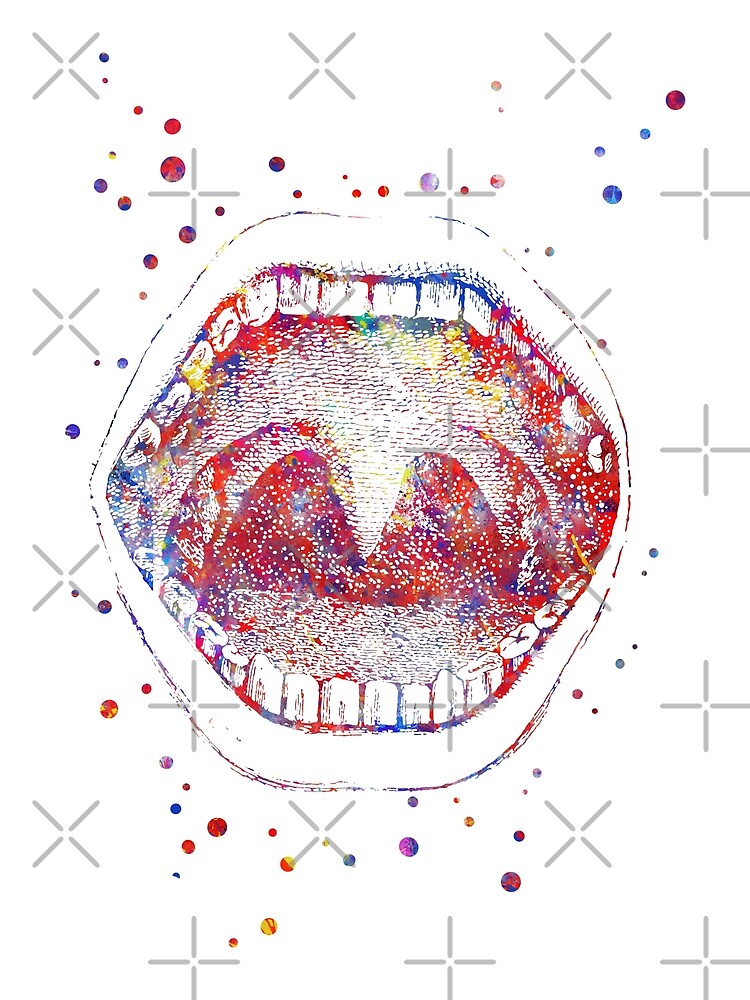The image is a detailed artistic representation of an open human mouth, rendered using digital graphic tools. The rectangular artwork lacks a definitive border or background, instead featuring a pattern of grey watermarks consisting of X's and plus signs spread across the image, likely to prevent unauthorized copying. The mouth is illustrated in such a way that you can see two rows of teeth, the tongue, and even the tonsils at the back of the throat. The interior is depicted with pixelated dots of various colors like purples, oranges, reds, and blues. Surrounding the mouth, the outer regions are filled with vibrant colored dots, some larger and multi-colored, adding to the artistic flair. Despite the detailed visualization of anatomical elements, it is impossible to determine the age or gender of the individual. This clip art, devoid of any text, serves as a visually striking piece that marries digital illustration with a colorful artistic approach.